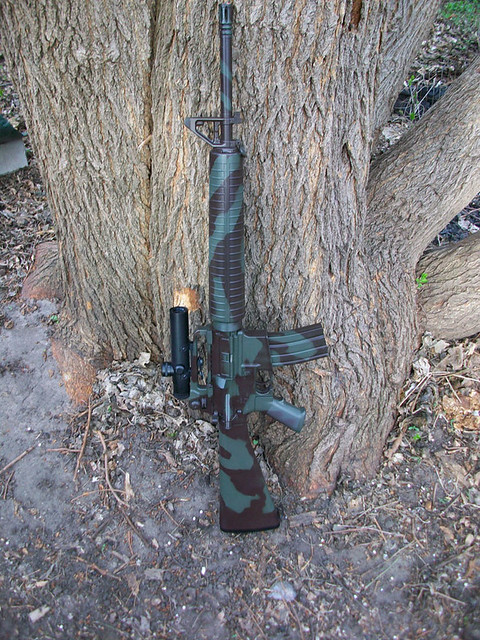The photograph captures a vertically oriented image of the base of an old, thick tree trunk with several split parts, primarily two main trunks extending vertically and two smaller branches stretching to the right. The ground is a grayish dirt surface, scattered with twigs, rocks, roots, and dead leaves, suggesting an outdoor setting. Leaned against the tree trunk is a large gun, possibly an assault rifle or a sniper rifle, characterized by a camouflage pattern of green, brown, and black hues. The gun is positioned vertically, with the stock resting on the ground and the barrel leaning against the tree. The weapon features a curved magazine protruding to the right, a grayish handle below it, and a ridged barrel that transitions into stripes matching the camouflage. Atop the gun, there is a black scope, adding to its detailed and formidable appearance.